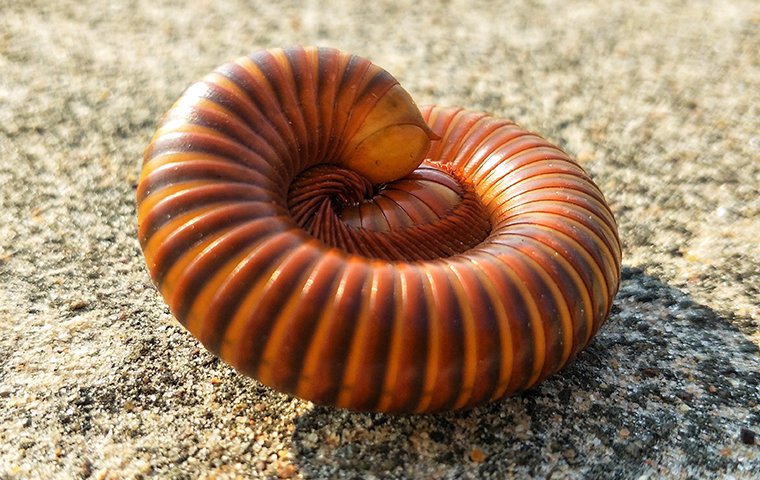This detailed photograph captures a curled-up centipede in the shape of a donut, basking in the sunlight on a sandy surface. The centipede is primarily brown with various shades of orange, and features distinct ridges and numerous legs, giving it a textured appearance. The sandy ground beneath it is a mix of light brown, black, and gray, with patches of green that hint at nearby vegetation or water. The sunlight illuminates the scene, casting shadows to the right of the centipede, and the background is slightly blurred, enhancing the focus on the intricate details of the curled-up creature.